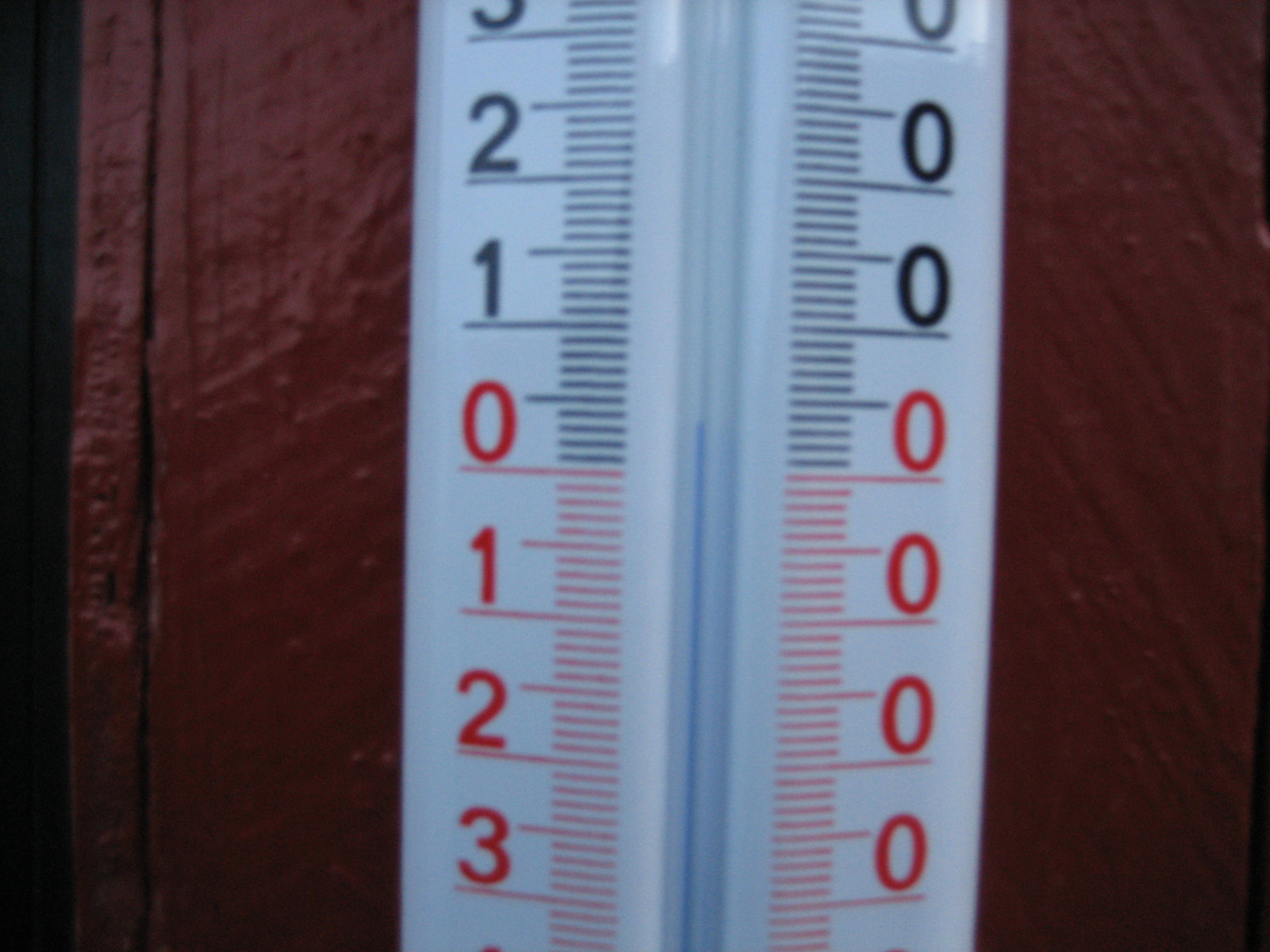In the photograph, a large, vintage-style outdoor thermometer dominates the frame, though part of it is cropped out. The thermometer is mounted on a surface that appears to be either a wooden post or wall, painted in a dark maroon color. At the center of the image is the white temperature gauge. The design features red numerals and markings on the lower half, while the upper half shifts to black numerals and lines.

On the left side of the gauge, the temperature markers include a red "0" at the bottom, ascending through "1", "2", and "3", with each numeral separated by short horizontal lines. Midway up the thermometer, the numbers change to black with a "1" at the center, above which are additional ascending numerals.

On the right side, the black numerals mirror the left, starting with "0" in the middle and aligning upward. Under these are four rows of black zeros. The mercury tube, or what appears to be a temperature-indicating fluid which is strikingly blue rather than the conventional red, hovers just above the zero mark. The detailed gradations of the gauge are visible, with each increment clearly delineated to provide precise temperature reading.

This particular aesthetic and placement suggest it may serve both functional and decorative purposes in a backyard or garden setting.